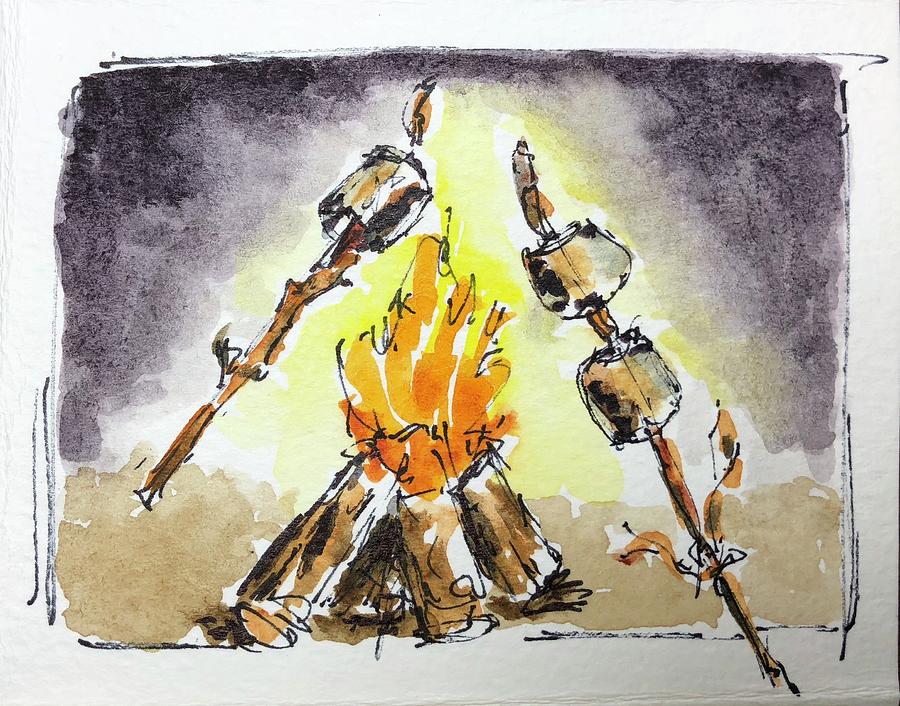The image appears to be a detailed drawing or watercolor on white paper, contained within a square outline. Central to the composition is a campfire, depicted with logs stacked on their sides, featuring brown hues interspersed with white highlights. The fire itself bursts forth in vibrant shades of orange, yellow, and touches of black, illustrating its dynamic flames. To the left of the fire, there is a stick emerging from the bottom left and extending upwards to the right, holding a marshmallow above the flames. Another stick, starting outside the square frame at the bottom and curving up to the left, holds two marshmallows; the top one positioned to the right of the upper part of the fire and the lower one near the bottom of the fire. The fire's glow is suggested by a yellowish hue that arches above and encircles the flames. The background is quite expressive: the upper corners blend gray and purple tones, while the bottom corners exhibit a brownish color, likely representing the ground the fire rests upon. The sky transitions from blackish and pinkish shades in the outer regions to yellow and white closer to the central fire, emphasizing the light it emits. There might be a signature or some marks near the bottom of the logs, and the bottom right-hand corner of the square contains small, illegible black writing.